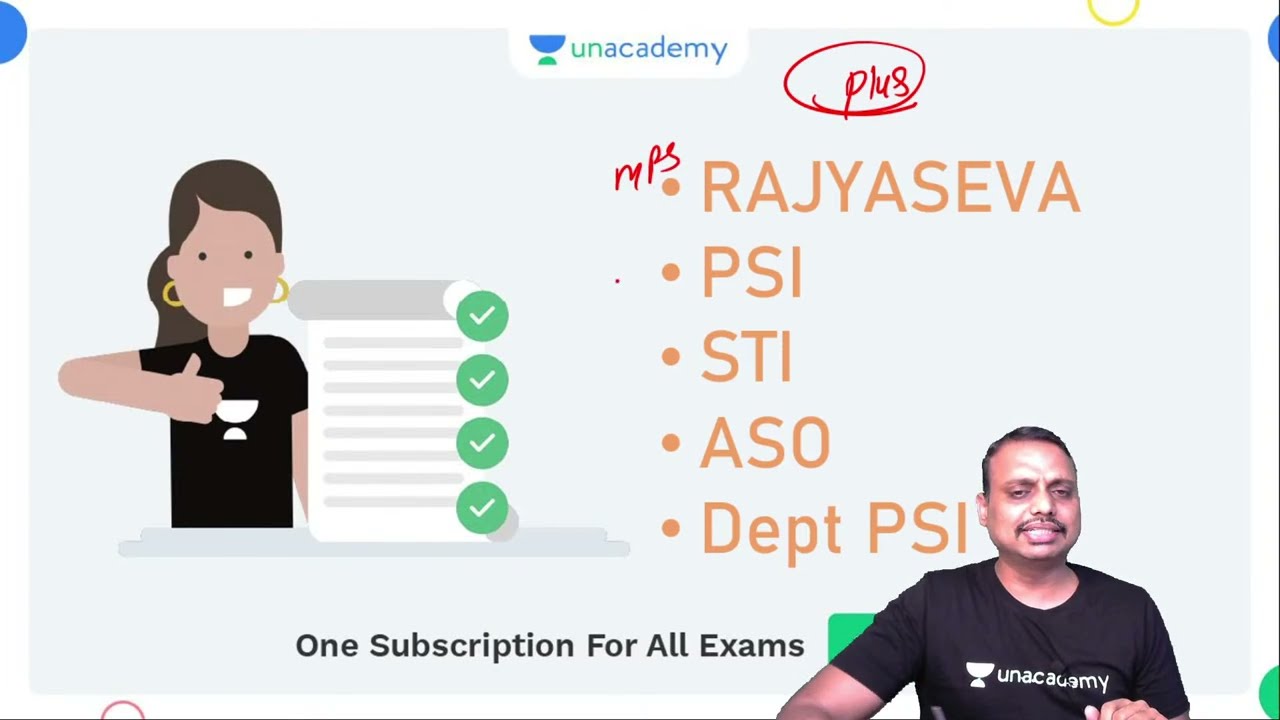The image showcases a promotional slide for Unacademy. Featured prominently in the bottom right corner is a man of Indian descent, sporting a short haircut, a mustache, and wearing a black short-sleeve shirt emblazoned with the Unacademy logo. He appears to be presenting or possibly live-streaming to promote the platform. A PowerPoint-like slide takes up much of the background, decked with various informative elements. Across the top is a header that reads "Unacademy," accompanied by a scribbled red "PLUS" symbol. Below, a list of bullet points includes "RANISFA," "PSI," "STI," "ASO," and "DEPARTMENT PSI." To the left of the center, an illustration of a woman with a ponytail, dressed similarly in a black shirt, is giving a thumbs up and smiling. In bold, black text at the bottom of the slide, it declares, "One subscription for all exams." The slide also incorporates a mix of colors, including black, white, gray, green, blue, yellow, brown, pink, and gold.